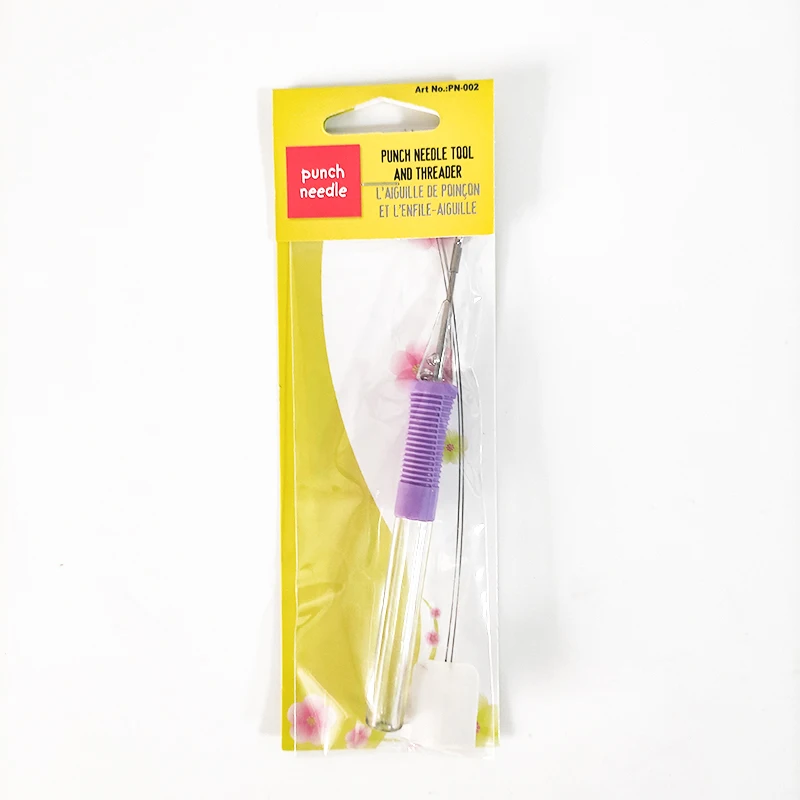The image depicts a product named Punch Needle, showcased against a very light beige or white background in a square-shaped, realistically taken photograph. The product is encased in a clear, vertically-oriented plastic sleeve, designed likely for display on a store shelf. The top section of the packaging features a yellow text box inscribed with "Punch Needle Tool and Threader" in black font. Directly to the left of this text box, a red square with the words "Punch Needle" in white font is prominently displayed. The logo is placed on the top left of the packaging. The visible Punch Needle Tool inside the plastic sleeve consists of a glass tube with a purple handle and a flexible plastic section positioned above the tube. Attached to the top of the device is a small metal pin, which is connected to two lines of thread extending upwards. At the end of one line, a tiny piece of paper can be observed. The background behind the product incorporates a subtle, sloping swirl design in yellow, adding an artistic touch to the packaging.